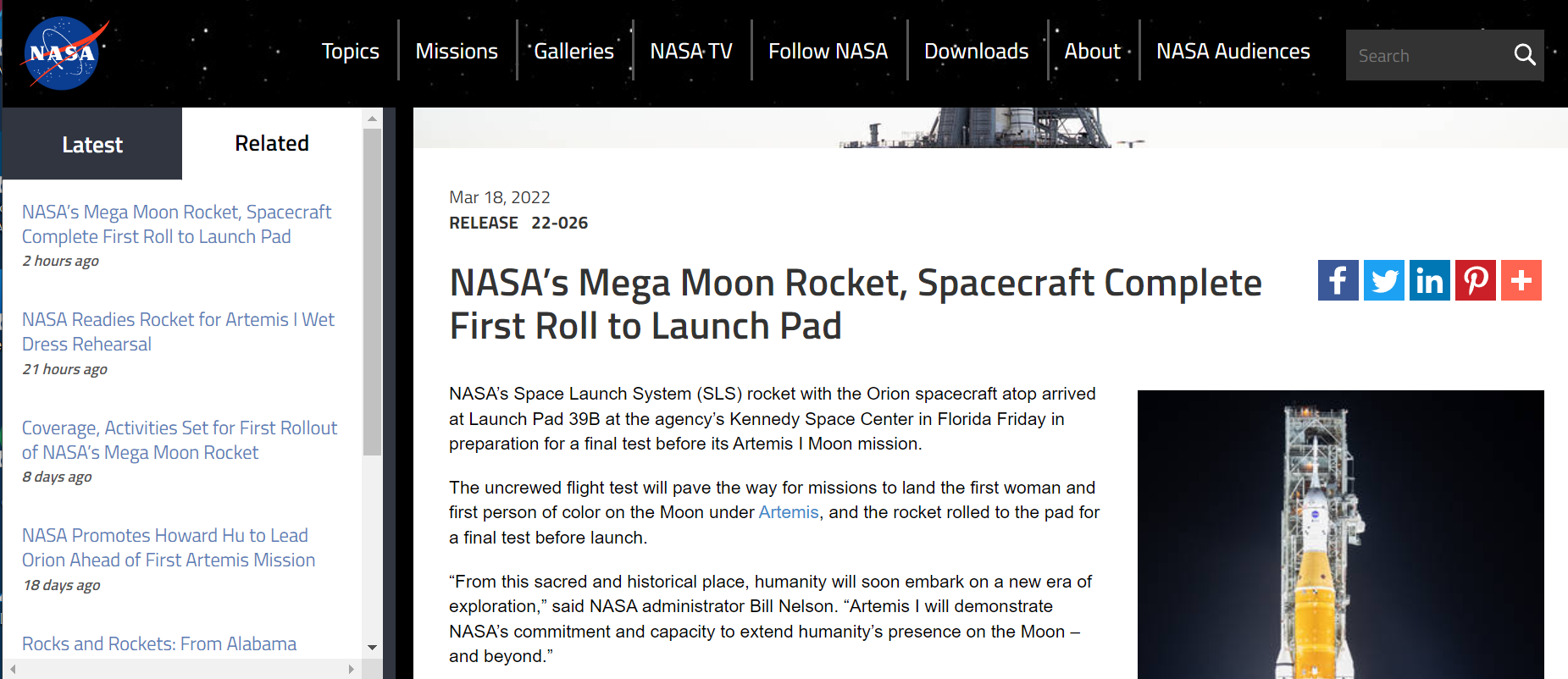Screenshot of NASA's Website Detailing the Artemis I Mission Preparations

This screenshot from NASA’s official website features a comprehensive layout detailing various updates and articles. On the left-hand side, the iconic NASA logo is prominently displayed. The logo features a blue Earth backdrop with the acronym "NASA" in bold letters and a red, forked-tongue symbol, often referred to as the "NASA red chevron."

Two main navigation tabs are visible at the top: "Latest" in bold white text against a dark gray background, and "Related" in bold black text on a white background. Below the tabs, several articles are listed as hyperlinked titles in blue text:

1. "NASA's Mega Moon Rocket, Spacecraft Complete First Roll to Launch Pad" - 2 hours ago.
2. "NASA Readies Rocket for Artemis I Wet Dress Rehearsal" - 21 hours ago.
3. "Coverage Activities Set for First Rollout of NASA’s Mega Moon Rocket" - 8 days ago.
4. "NASA Promotes Howard Hu to Lead Orion Ahead of First Artemis Mission" - 18 days ago.
5. "Rocks and Rockets from Alabama."

A gray bezel on the right side houses several widgets. Towards the bottom, there is a medium gray section with a dark gray rectangle inside it. The top portion features a black bezel adorned with white dots representing stars. Several white clickable tabs, separated by thin white lines, include categories such as "Topics", "Missions", "Galleries", "NASA TV", "All of NASA", "Downloads", "About", and "NASA Audiences".

The dark gray search bar situated on the right-hand side contains lighter gray text that reads “Search” and is accompanied by a white magnifying glass icon. Below, an image captures a space shuttle poised against a gleaming silver launch pad. The shuttle is primarily white with an orange base, accentuated by bands of yellow and white. At the top left of the image, the date "MAR 18, 2022" is indicated, followed by the release code "2022-026" in bold black text.

Adjacent to the image, the headline "NASA’s Mega Moon Rocket, Spacecraft Complete First Roll to Launch Pad" is showcased in bold black text. Aligned to the far right of the page, a series of social media buttons are arranged: 

- Dark blue with a white "F" for Facebook
- Medium blue with a white bird for X (formerly known as Twitter)
- Dark blue with a white "I" for LinkedIn
- Dark red with a bold white "Q" for Pinterest
- Orange with a white plus symbol, possibly for adding further social media options.

Below the headline, a detailed paragraph summarizes the event: "NASA's Space Launch System (SLS) Rocket with the Orion spacecraft atop arrived at launch pad 39B at the agency's Kennedy Space Center in Florida Friday in preparation for the final test before the Artemis I moon mission." 

A new paragraph highlights the mission's significance: "The uncrewed flight test will pave the way for missions to land the first woman and first person of color on the moon under Artemis," with a hyperlink provided for further information. The paragraph continues: "The rocket rolled to the pad for the final test before launch."

Quotations from NASA Administrator Bill Nelson are included: "From this sacred and historical place, humanity will soon embark on a new era of exploration," and, "This Artemis I will demonstrate NASA’s commitment and capacity to extend humanity’s presence on the moon — and beyond."

This detailed screenshot effectively encapsulates NASA's recent updates and ongoing preparations for the Artemis I mission.